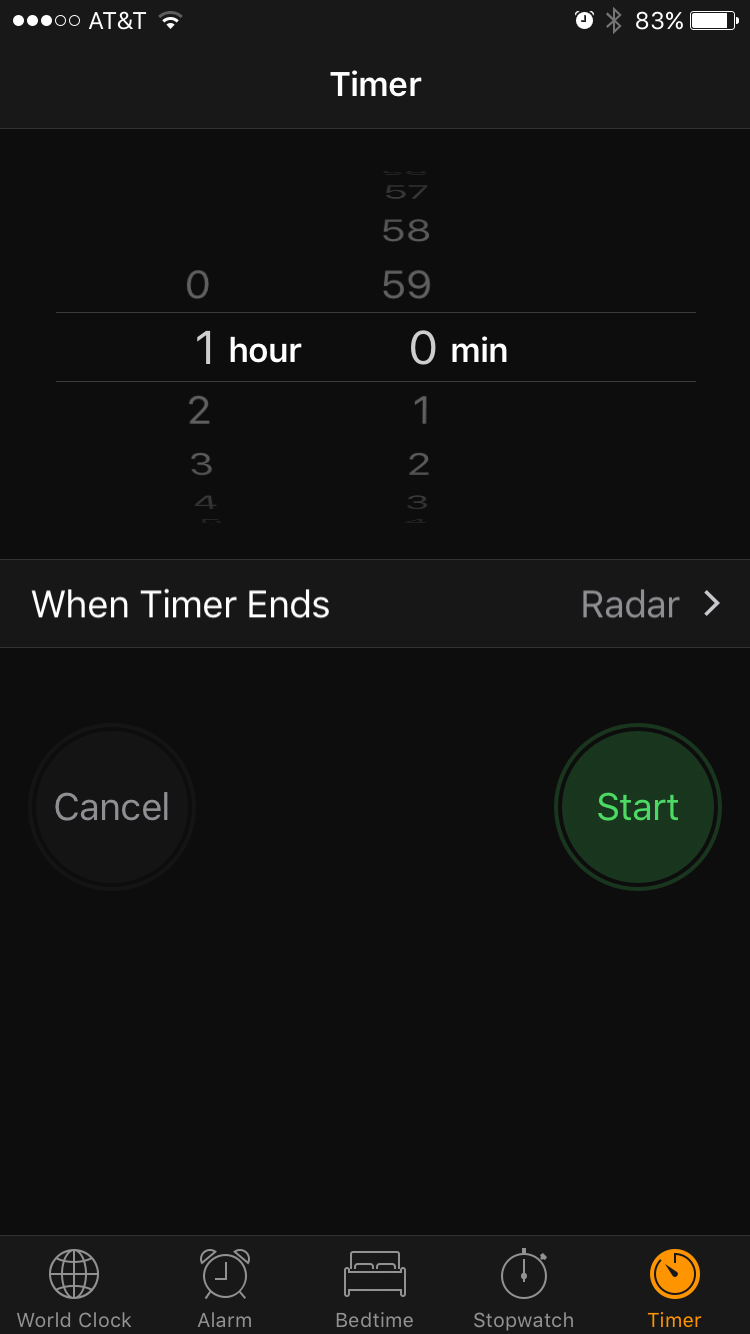A detailed online interface screen features a shadow box message at the top left reading "Flag as inappropriate." The user is currently utilizing an ATM, indicated in the top-left corner. The interface has a black background with white text, highlighted by a green "Start" button on the right side and a gold clock icon at the bottom right. The battery level at the top right shows 83%. Centrally located near the top, the screen displays "Timer" with "One hour and zero minutes" prominently highlighted in white. Below, it states "When timer ends, radar indicator" in white text on the black background. To the left of the green "Start" button, there's a black "Cancel" button with white text. At the very bottom of the screen are several icons: a globe for the world clock, an alarm clock for alarms, a bed for bedtime, a stopwatch for the stopwatch function, and farthest to the right, a goldish-orange timer icon.